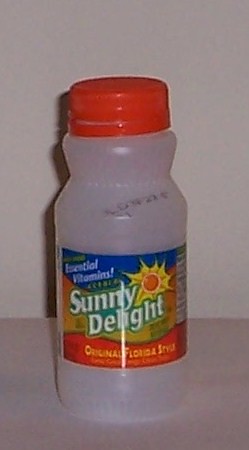This image showcases an empty plastic bottle of Sunny Delight set against a clean, white background. The bottle features an orange twist-on cap and sits on a slightly darker gray surface. The label on the bottle is vividly detailed: the prominent Sunny Delight logo is in white lettering with a green outline, standing out against a gradient label background that transitions from blue at the top, to yellow in the middle, and dark orange at the bottom. To the top left of the logo, the words "Essential Vitamins" are displayed in white text on a blue background, accompanied by a sun graphic on the right. Below the Sunny Delight logo, the phrase "Original Florida Style" appears in bright orange lettering on the dark orange section of the label. Despite the small, hard-to-read expiry date near the cap, the nutritional facts are also visible but somewhat obscured due to the angle. A distinct shadow behind the bottle and a central line of reflection hint at the bottle's curvature and transparency.